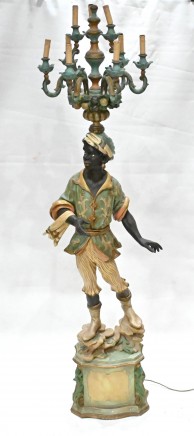This portrait-oriented photograph features a meticulously detailed figurine set against a slightly crumpled cloth background, giving the scene an elegant yet antiquated ambiance. The focus is on a sculpted ornament, possibly made of clay and finished to a solid form, standing on a bronze base with greenish and yellow patina that evokes an aged appearance, as if it had been exposed to the elements.

The figurine portrays an individual with nearly completely black skin, adorned in richly textured attire. The figure sports gold boots atop the bronzed base, adding to the regal aesthetic. They wear three-quarter length stripy trousers that resemble corduroy and flare out at the knees, paired with a flared, buttoned green top adorned with silvery gold swirls. The short-sleeved top has voluminous sleeves that almost appear bagel-like around the arms.

In a poised stance, the figure's right arm is bent at the elbow, holding a folded tea towel or napkin over the crook. The left hand is slightly extended away from the body at a 45-degree angle. Atop the figure’s head is a visually striking lamp, designed like a candelabra with multiple U-shaped arms, each holding a candle. The candelabra, crafted from greenish metal with bronze tinges, features two tiers: the lower tier with four candles and the upper tier with two, creating a symphony of light that crowns the figurine. Completing the ensemble, the individual wears a green hat with a gold band encircling it.

The pedestal on which the figurine stands appears rocky and aged, harmoniously matching the candelabra's patina. The entire setup, though seemingly indoor, conveys an outdoor relic's timeless charm.